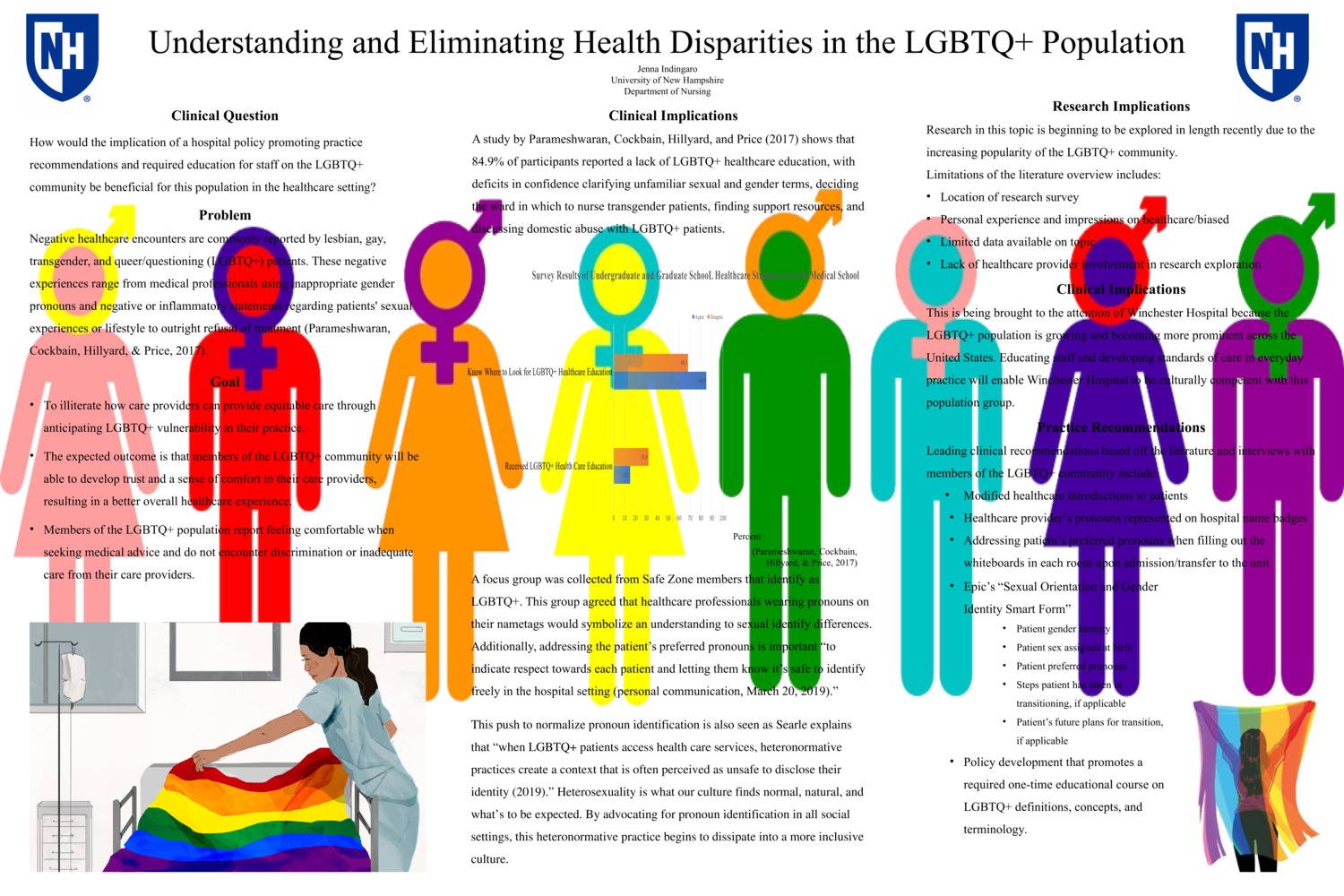This image features an informational poster titled "Understanding and Eliminating Health Disparities in the LGBTQ Plus Population." In the top corners, there are logos of a blue shield split with blue and white letters "NH," representing New Hampshire University. The poster consists of three columns of text under the headings: Clinical Questions, Clinical Implications, and Research Implications, each containing several paragraphs of detailed information.

Dominating the center are colorful generic human figures in pink, red, orange, yellow, green, blue, indigo, and purple, each with different gender symbols as their heads, reflecting diverse gender identities. 

On the upper left, a cartoon nurse is seen making a hospital bed with an LGBTQ+ rainbow blanket, and in the lower right, there is a silhouette of a female figure holding an LGBTQ flag. These visual elements serve to emphasize the inclusivity and focus of the poster on LGBTQ+ health disparities.